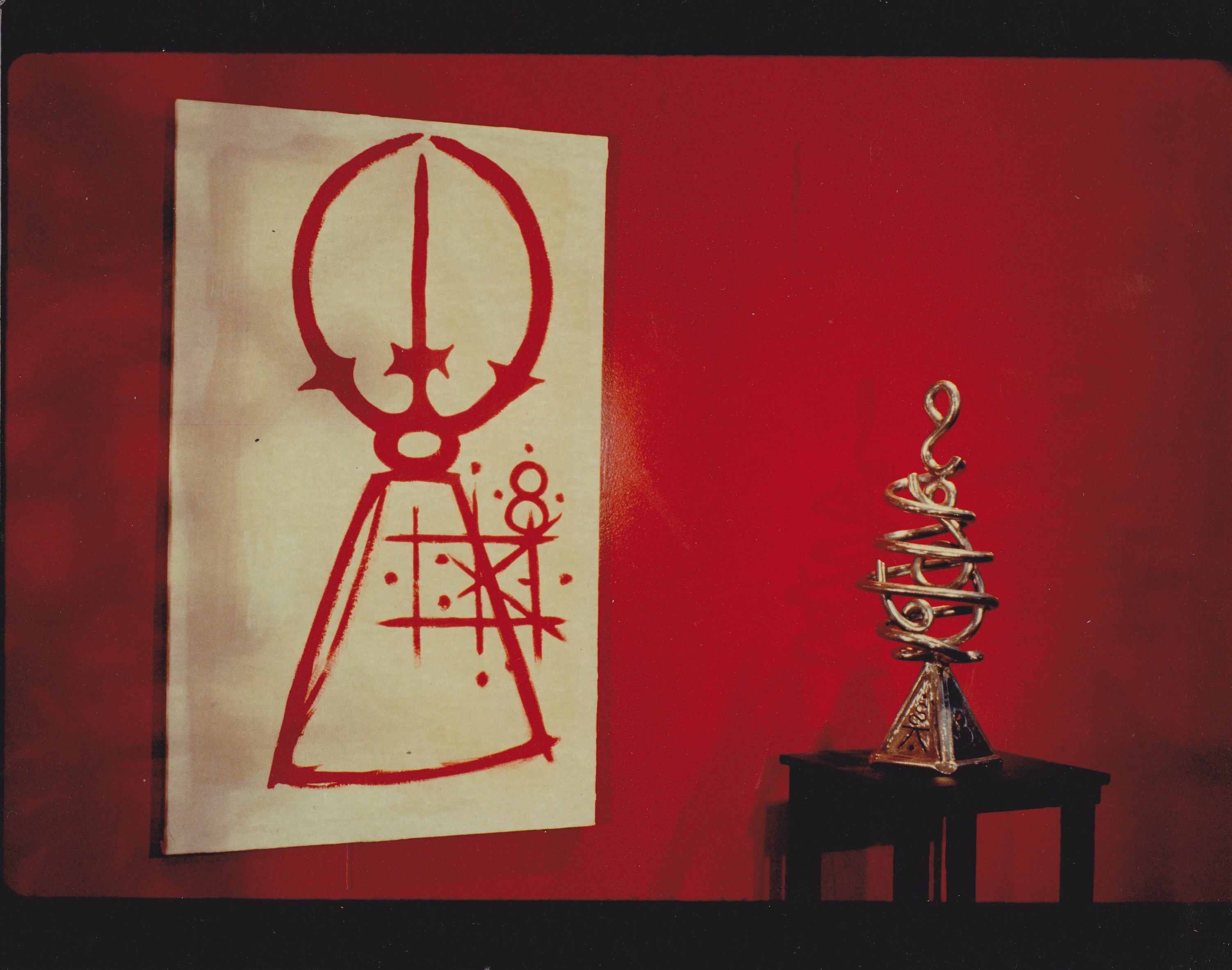In this realistic painting, a small black table with a triangular base, adorned with intricate spirals and loops, supports an ornamental gold sculpture. Resembling abstract symbols or possibly even a ship anchor or fishhook, this metallic piece swirls upward in a strikingly modern and elaborate design. The sculpture is set against a vivid red wall, intensifying the visual boldness of the scene. On the left side of the composition hangs a white banner featuring red line drawings, including a circle with a sword, a cone design, and several cryptic symbols, exuding a mysterious, almost cult-like aura. The meticulous shadows cast on the red background further enhance the realism and depth of the painting.